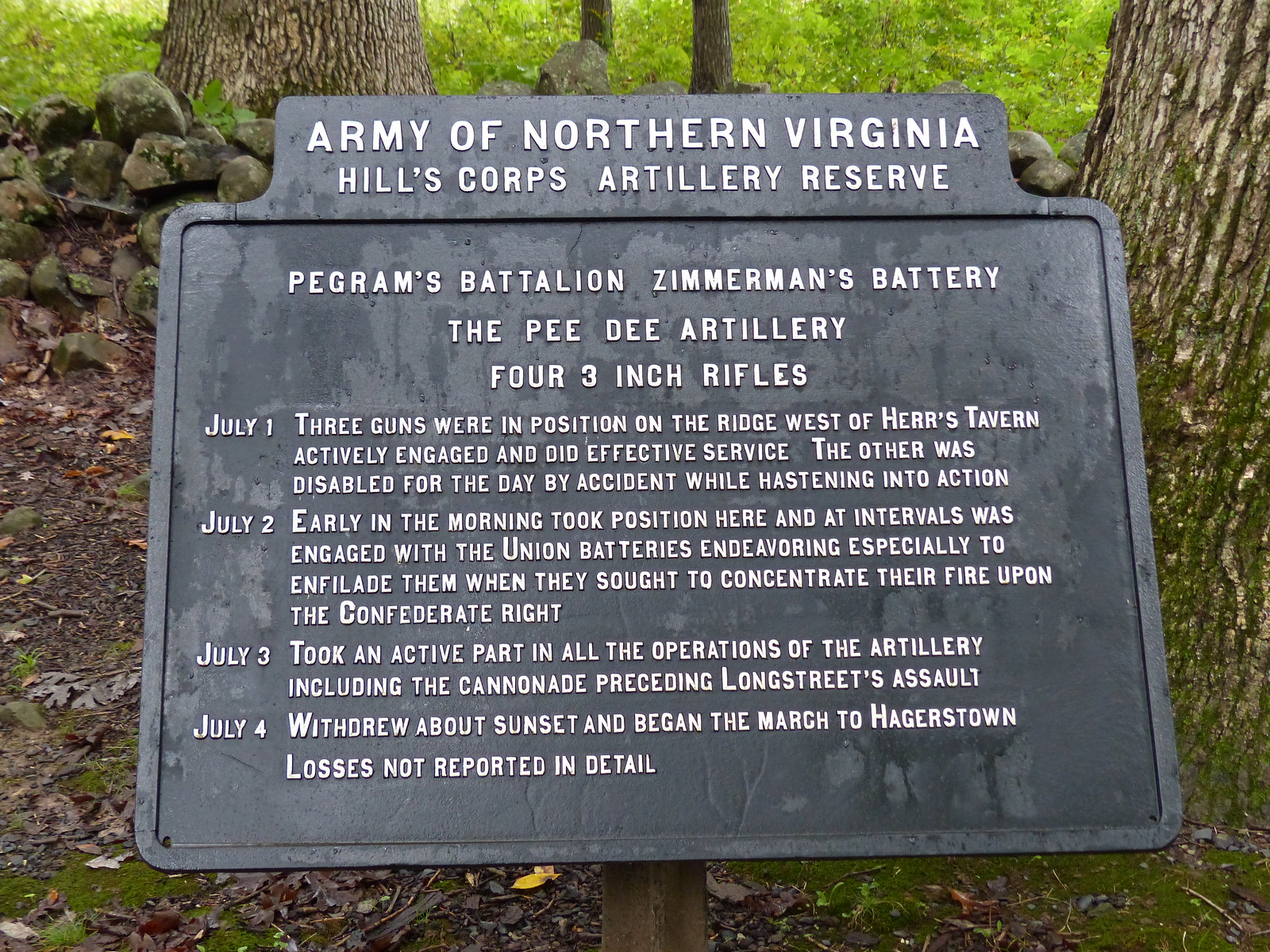The image features a clean, recently rained-on black plaque situated at a historical memorial site with trees, grass, and a small stone wall in the background, suggesting it was taken in spring or summer. The plaque, adorned with white text, is titled "Army of Northern Virginia, Hill's Corps Artillery Reserve." Below this, in smaller white font, it reads "Pegram's Battalion, Zimmerman's Battery, the P.D. Artillery, Four Three-Inch Rifles." The plaque details events from July 1st to July 4th:

- **July 1st:** "Three guns were positioned on the ridge west of Herr's Tavern, actively engaged, and did effective service. The other was disabled for the day by accident while hastening into action."
- **July 2nd:** "Early in the morning, took position here and at intervals was engaged with the Union batteries, endeavoring especially to infilate them when they sought to concentrate their fire upon the Confederate right."
- **July 3rd:** "Took an active part in all the operations of the artillery, including the cannonade preceding Longstreet's assault."
- **July 4th:** "Withdrew about sunset, and began march to Hagerstown. Losses not reported in detail."

This meticulously maintained memorial plaque serves to commemorate the engagements and movements of Pegram's Battalion during this critical period.